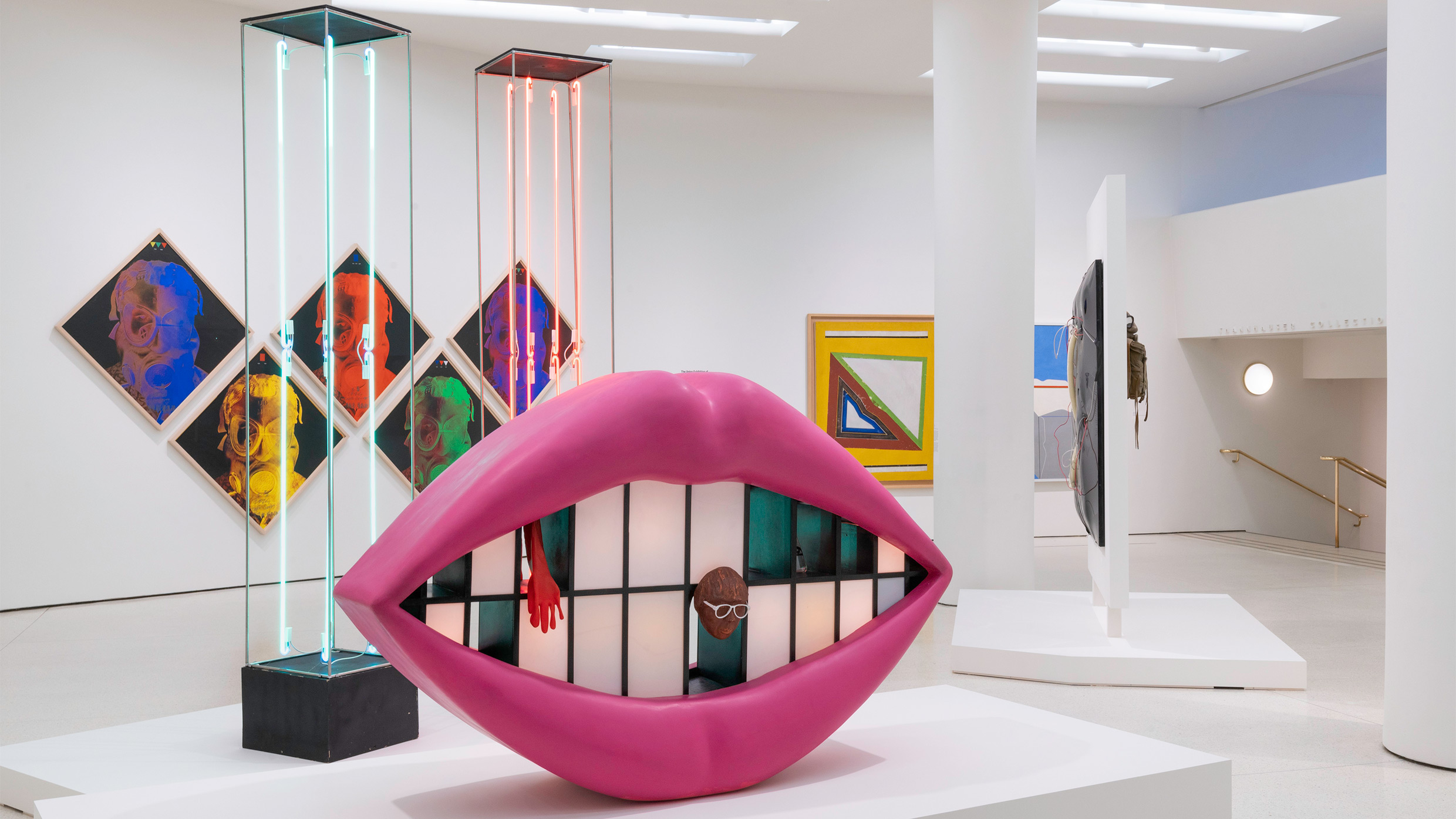The photograph captures a striking scene inside a modern art museum, where the austere white walls, ceiling, and flooring provide a stark backdrop for the colorful installations. Center stage is a large, eye-catching sculpture of bright pink lips, which is adorned with white teeth, including some that are missing. Intriguingly, a human head protrudes from one of the gaps, while a hand emerges from another. Just behind this central piece stand two tall neon pillars, one glowing with red light and the other with blue.

The background features five diamond-shaped paintings arranged in a single row, each in a distinct color: purple, yellow, red, green, and another shade of purple. The effect is a vibrant spectrum set against the pristine white surroundings. Additional paintings can be seen on the walls, although their details remain less distinct. To the right, a brass staircase with golden handrails descends, adding a touch of elegance to the contemporary setting. The space is bathed in a palette that includes pinks, blues, yellows, oranges, greens, and purples, combining to create an aesthetically rich environment.